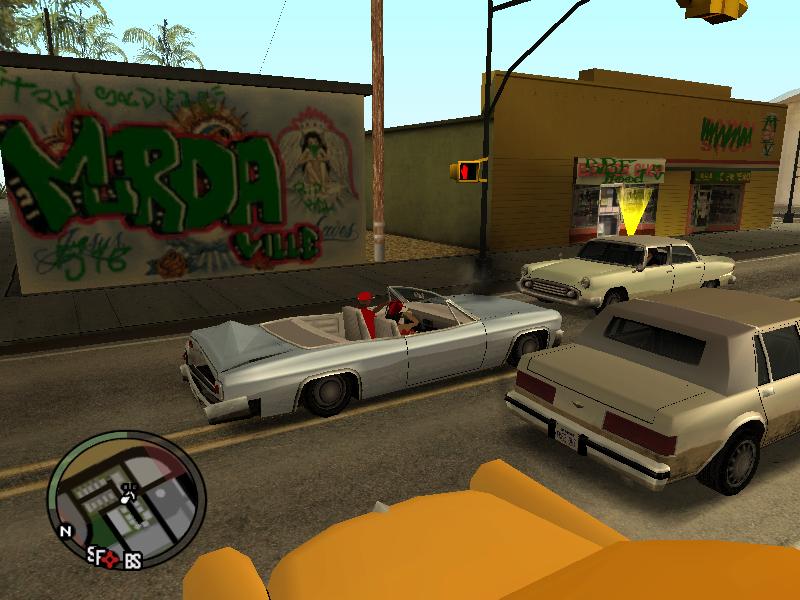The image resembles a snapshot from a video game, set in a quaint, slightly rundown small town. Several vehicles are visible on the road, including a notably dilapidated silver sedan with a soft top, marred by extensive rust. Along the curbside, a building covered in numerous graffiti tags stands out, symbolizing the town's gritty character. Adjacent to this graffiti-laden structure, there's a slightly upscale building that appears to be a restaurant, adding a touch of contrast to the scene.

Among the vehicles, a man in a red shirt and matching red cap is seen driving a silver convertible with the top down, cruising leisurely through town. Meanwhile, a pristine white sedan, reminiscent of an old Mercedes, is either parked along the curb or navigating in the opposite direction, adding a classic charm to the otherwise rugged setting.